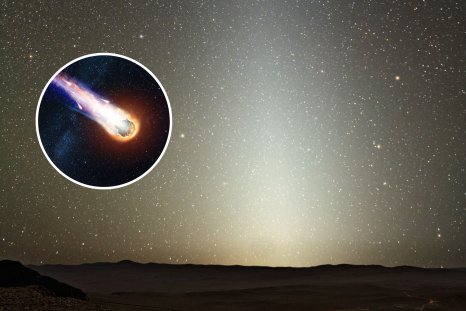This textbook-style photograph captures a vividly illuminated night sky brimming with countless stars, set above a slightly uneven, hilly terrain at the bottom of the image. Dominating the center of the scene, a bright light rises from the horizon, casting a faint glow yet still allowing the stars to sparkle through. To the left, nearly central in the image, there's an inset circle outlined in white, depicting an artistic representation of a comet. This comet is shown as a round object with fire flaming behind it, in striking hues of golden, white, and purple, giving the impression of momentum across a dark, star-studded background. The overall composition appears ideal for educational purposes in science textbooks, focusing on celestial phenomena like stars, the night sky, and especially comets.